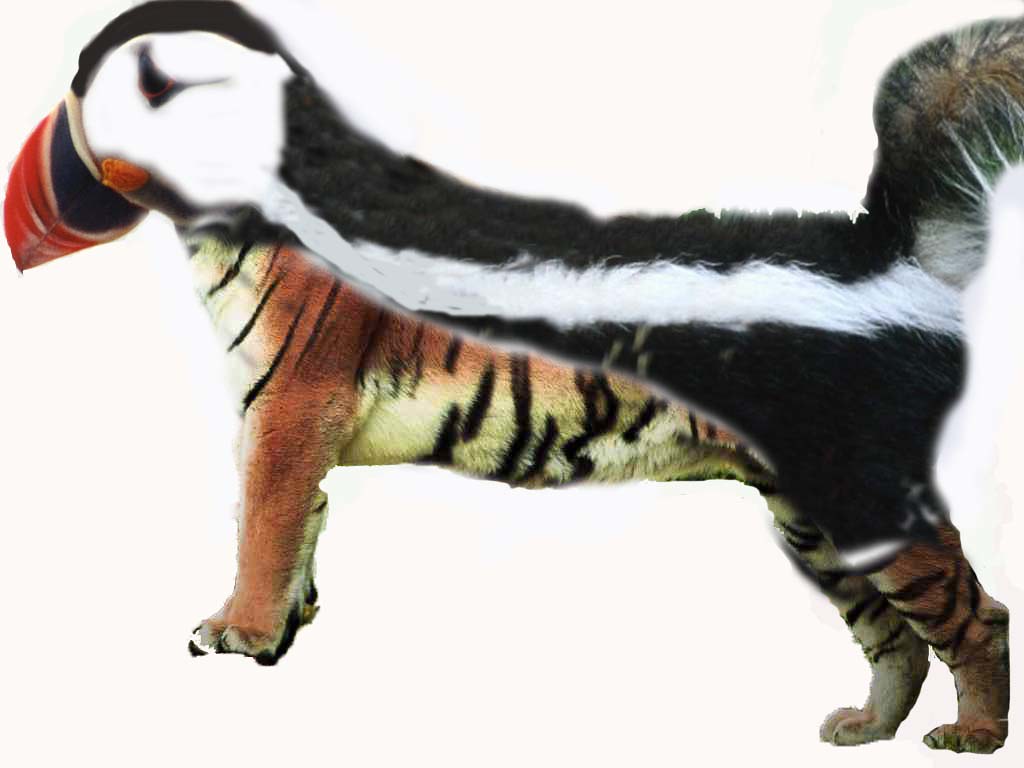The image showcases an AI-generated hybrid animal, combining features from multiple species, set against a white background. The creature's head resembles that of a parrot, with a distinct red beak and a predominantly white face topped with black. The upper part of the body is reminiscent of a skunk, featuring a black coat accented by a prominent white stripe running along its back. The animal's tail is bushy, akin to that of a squirrel or skunk. The lower body and all four legs exhibit characteristics of a tiger, with orange fur and black stripes, complemented by white tufts of hair. The overall effect is a surreal amalgamation of various animal parts, creating a fantastical and bizarre entity.